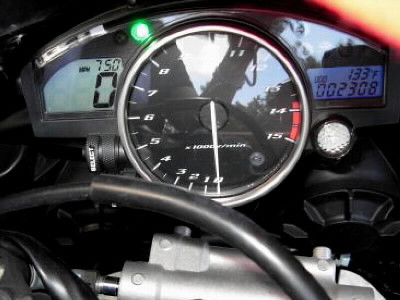The image depicts an intricate component inside a vehicle, showcased with meticulous detail. At the center of focus is a prominent silver casing surrounded by a network of black hoses. Above this, a large, round gauge numbered from 0 to 15 is prominently displayed. The gauge’s face is black with white numerals, where the scale starts at 0 at the 6 o'clock position and ascends clockwise to 15 at the 4 o'clock position. The numbers 14 and 15 are highlighted in a red zone, indicating a critical range. The needle, however, is currently pointing downwards at 0. 

To the immediate right of the dial gauge is a digital meter displaying the number "0". Above this, in smaller lettering, it reads "750" followed by an abbreviation that seems to be "MGM" or something similar, the exact letters being unclear. Further to the right, there is a small silver button which is situated beneath another gauge. This gauge shows a reading of "133 degrees Fahrenheit" and below this, a numerical sequence "002308" is displayed. The complex setup suggests the gauges are likely measuring various parameters such as speed and temperature, possibly within a specialized vehicle or machinery context.